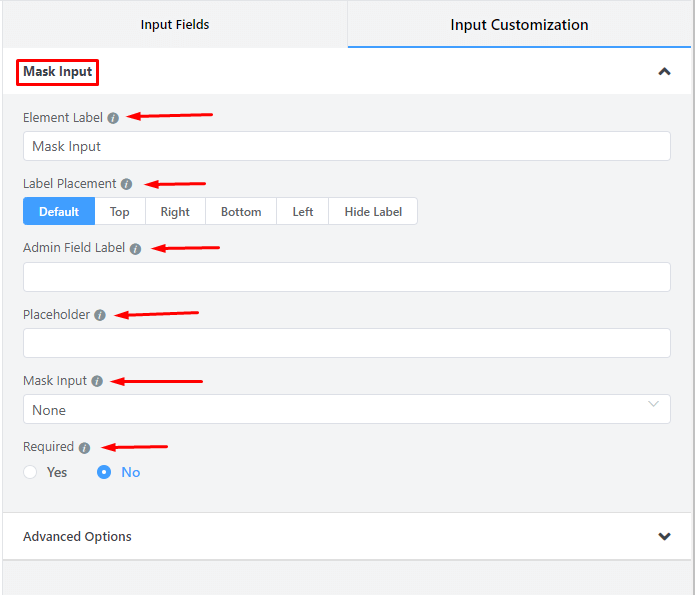A desktop screenshot displays an interface predominantly set against a light gray background with elements of white. In the top left corner, "Input Fields" is prominently labeled, with "Input Customization" selected, distinguished by a thin blue line underneath.

Below "Input Fields" on the left, "Masked Input" is highlighted with a red rectangle, and to its extreme right is an upward-facing arrow. Adjacent and slightly below "Masked Input" is "Element Label," noted with a red arrow pointing towards it. Directly under this label, a white input field displays the text "Mask Input."

Further down, "Label Placement" is labeled, accompanied by a red arrow. It includes several tabs: "Default," marked by a blue rectangle indicating its selection, followed by "Top," "Right," "Bottom," "Left," and "Hide Label."

Continuing downward, "Admin Field Label" is indicated with another red arrow, followed by an empty white rectangular input field. Below this, "Placeholder" has a red arrow pointing to it with an accompanying input field underneath. Below the field, "Mask Input" again features, marked with a red arrow directing to a search or input field labeled "None," which intriguingly has a dropdown button on its right side.

Towards the bottom, the term "Required" is mentioned alongside two radio buttons labeled "Yes" and "No," with "No" being selected. Finally, at the very bottom of the interface, "Advanced Options" is listed, featuring a dropdown button to its far right.